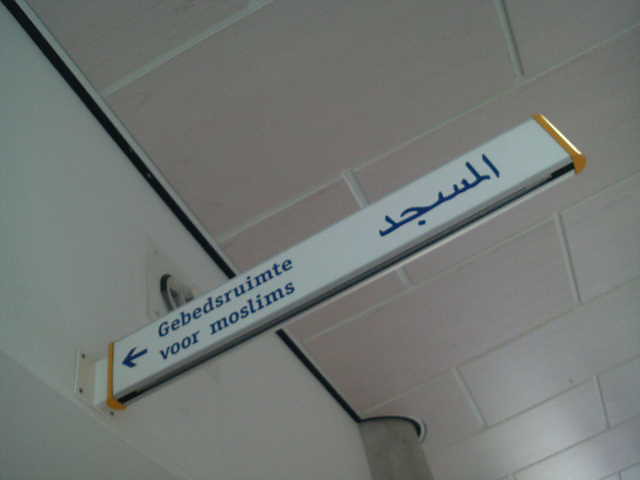The image showcases a distinctive sign protruding from a white tiled wall, viewed from a lower angle looking upwards. The sign, positioned diagonally from the lower left to the upper right, features bold blue lettering on a white background and has yellow end caps at both its attachment point to the wall and its opposite end. Above the sign, the white ceiling appears to be constructed from individual tiles. On the left side, the white wall includes a circular embedded feature above the sign. Additionally, a pole is mounted to the wall, extending vertically at the center-bottom of the frame.